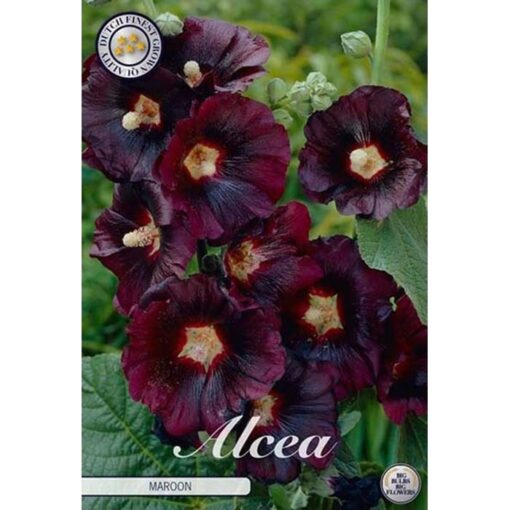The image showcases a close-up of ten azalea flowers in full bloom. The flowers exhibit a rich spectrum of dark purple to dark purplish-red hues, with some flowers featuring centers of light gold. Prominent green leaves with detailed veins surround the flowers, contributing to the bright green backdrop of the image. While most flowers are in full bloom, a few stems in the background reveal small green buds, suggesting some florals have yet to open. At the bottom middle of the image, the word "azalea" is printed in italics, while "maroon" is written in the bottom left corner. The top left corner features a circular logo stating "Dutch Finest Growing Quality" with five stars in the center, and the bottom right corner displays another circular logo with blue lettering.